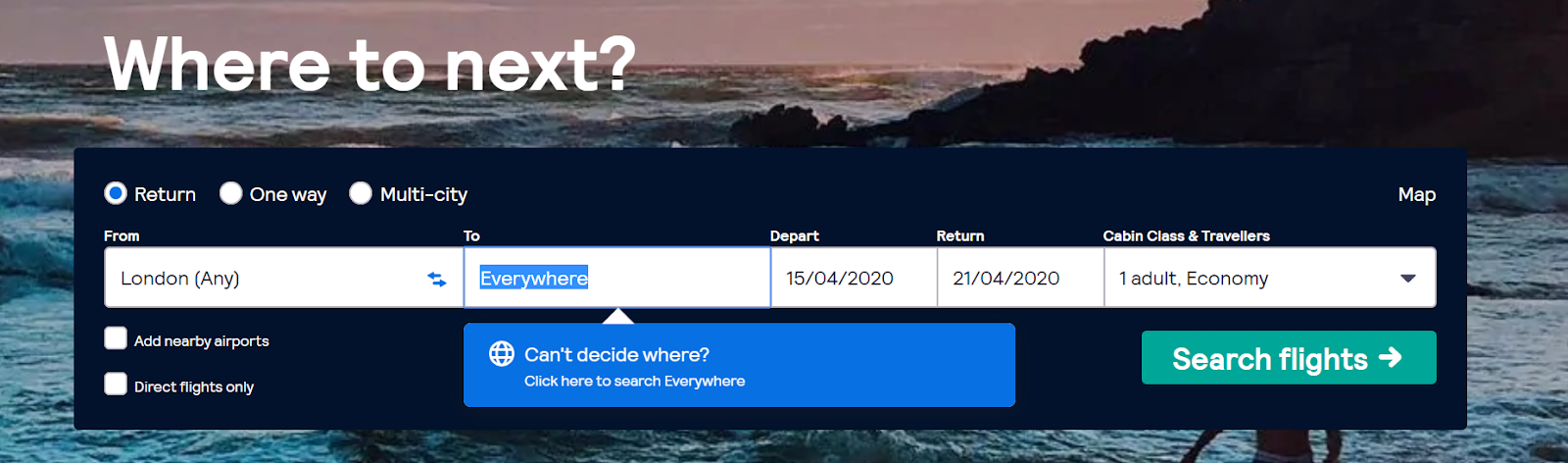In the image, there's a picturesque coastal backdrop featuring waves crashing against a rocky shore with a vast coastline extending into the distance. The scene is viewed from a wide-cropped angle, showing the back of an individual standing near the water, seemingly lost in contemplation. Superimposed on this tranquil setting is an interactive travel booking interface. The interface displays a search bar where "London" is entered as the departure location, with the destination set to "Everywhere." A dialogue bubble prompts the user, stating, "Can't decide where? Click here to search everywhere." Details for a trip are specified, with departure on April 15, 2020, and return on April 21, 2020, for one adult in economy class. A "Search Flex" button is prominently featured, suggesting a flexible search option. This innovative feature appears to cater to spontaneous travelers who are open to exploring various destinations without a fixed plan, making it a perfect tool for adventurous souls who prioritize the journey over the destination.